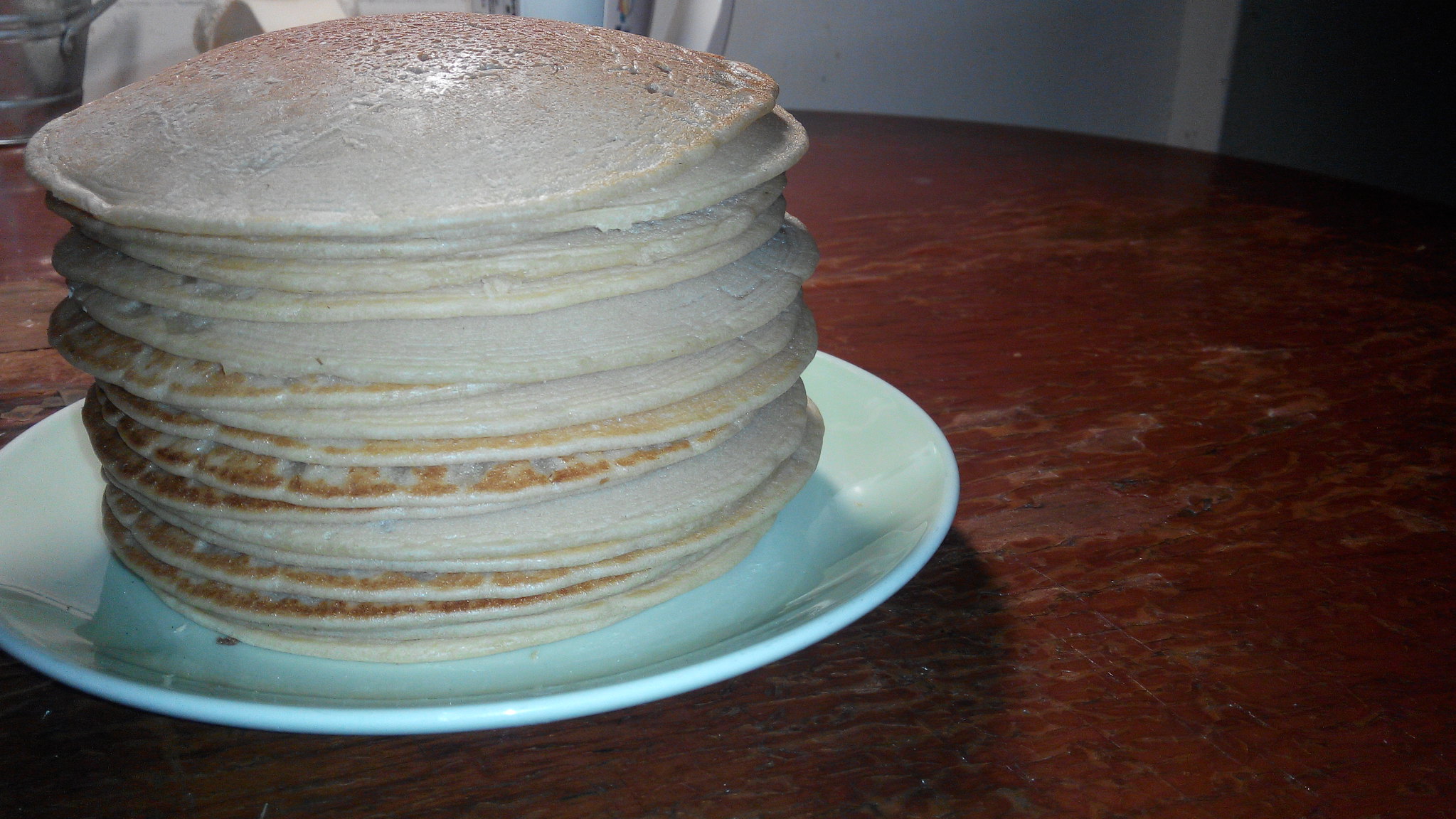The image features a slightly dark scene, likely taken in a dimly lit room with a flash, evident from the glare on a metallic handle in the top left corner of the frame. Dominating the shot is a large, round wooden table with a dark reddish-brown hue, marked with signs of wear and stripped paint. Positioned on the left side of the table is a light powder blue, bowl-like porcelain plate. This plate holds a tall stack of approximately 15-20 pancakes, which are predominantly pale and light brown, with some edges showing signs of browning, suggesting they may not be entirely cooked. The background reveals a greyish-beige wall, contributing to the muted ambiance of the scene.